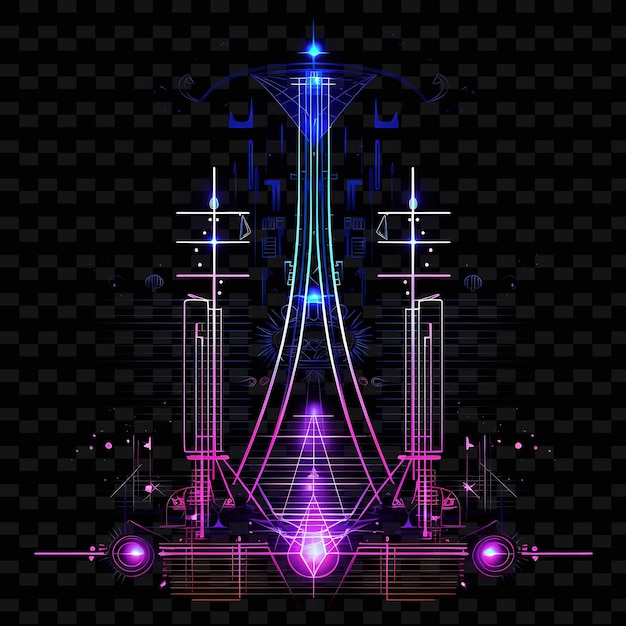This digital art piece features a central obelisk-like structure, reminiscent of the Eiffel Tower, rendered in vibrant neon colors against a black and dark gray checkered background. The tower rises from a pink teardrop shape at the bottom and transitions through purple, white, and light blue before culminating in a glowing blue star at the peak. Symmetrically flanking this central tower are two smaller spires, which also transition from pink to white, each adorned with three horizontal lines. At the base of the tower, there are two purple circular motifs on either side of the teardrop, intersected by horizontal purple lines. The entire composition is intricately detailed, with numerous lines and geometric shapes that enhance its futuristic, Art Deco-inspired aesthetic. The combination of glowing neon hues—pink, purple, blue, teal, and white—against the dark background gives the artwork a vibrant, electric feel, heightened further by its symmetrical, almost mirror-like arrangement.